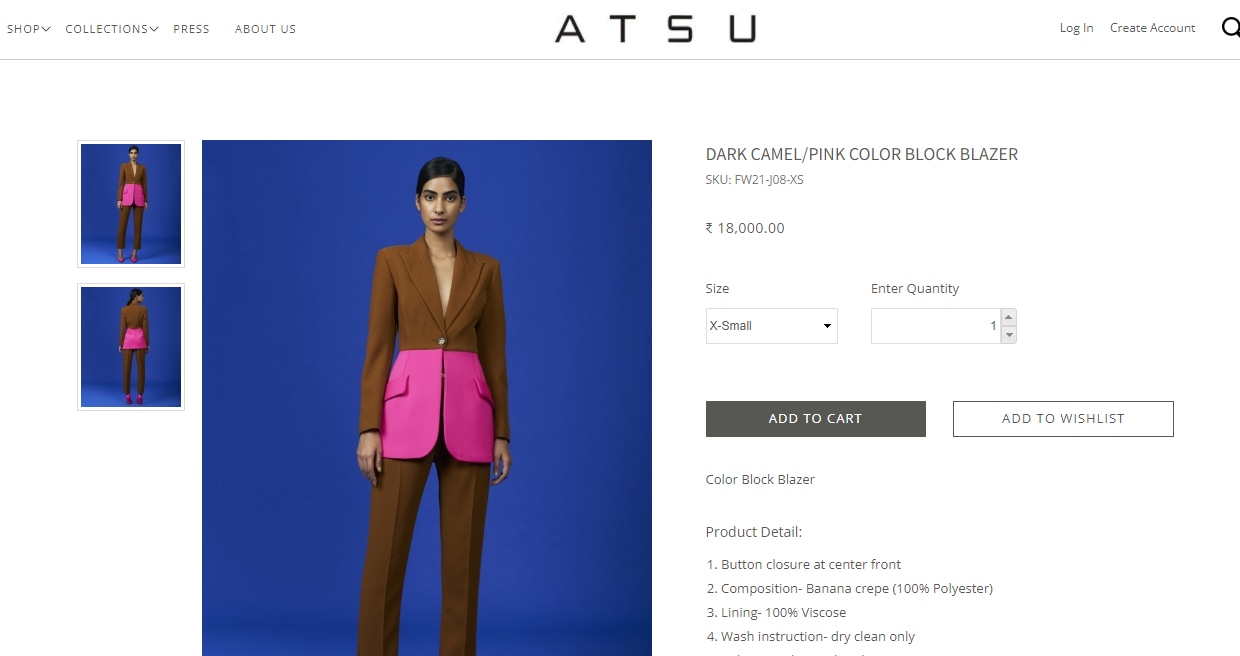Screenshot of a high-end women's fashion website with a sleek, minimalist design and a white background. At the top left, there's a clean four-label menu in gray with "Shop" and "Collections" having down arrows, while "Press" and "About Us" are plain. Centered on the page are large, bold black letters spelling "ATSU," the website's name. On the top right, it displays options in gray for "Log in," "Create Account," and a black search icon. 

Below the site name is a thin light gray line. On the left side of the page, there is a large image with a blue background showcasing an androgynous person with black hair, who is tall and slim. They're wearing stylish brown slacks and a unique, fashion-forward one-button blazer. The blazer is brown on the top half and sleeves, while the bottom areas, including the pockets, are pink. The blazer has a plunging neckline, as it's worn without a shirt underneath. There are two thumbnail images on the left showing back and full views of the outfit, including the feet and shoes.

On the right-hand side of the image, detailed product information is displayed. In light gray lettering, it reads "Dark Camel/Pink Color Block Blazer," along with a SKU number and a price marked in a foreign currency symbol as $18,000. Below this, there is a size selection window with "Extra Small" currently selected, alongside a drop-down arrow to choose different sizes. There's also an "Enter Quantity" section with 1 selected, and up and down arrows to adjust the quantity.

Further down, two horizontal buttons are displayed. The left button is dark gray with white lettering that says "Add to Cart," while the right button is white with gray lettering reading "Add to Wishlist." Underneath the "Add to Cart" button, the product details are listed as follows:
1. One-button closure at center front
2. Composition: Banana Crepe - 100% Polyester
3. Lining: 100% Biswa
4. Wash Instruction: Dry clean only.